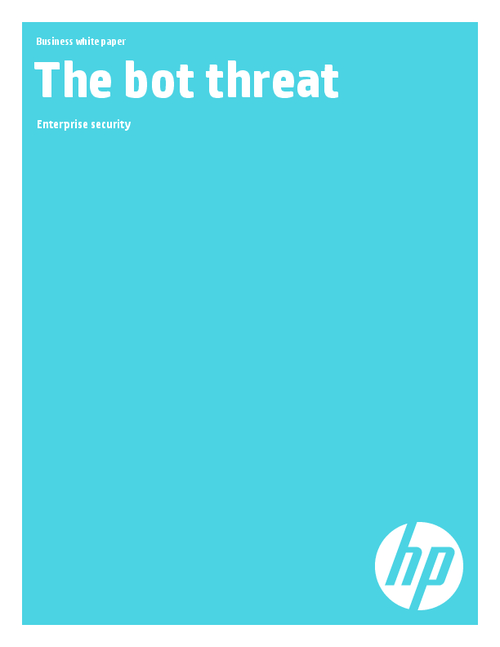The image displays a computer-generated, vertically-oriented graphic with a light blue background. At the top left, the white text is organized into three left-aligned rows: "Business White Paper" in a smaller font, "The Bot Threat" in bold and larger font, and "Enterprise Security" in a smaller font. The text is simple, with only the initial letters of each main word capitalized. In the bottom right corner, there is a white HP (Hewlett-Packard) logo. The overall design is minimalist, with ample empty space around the centered text and the logo, emphasizing the title and purpose of the document.